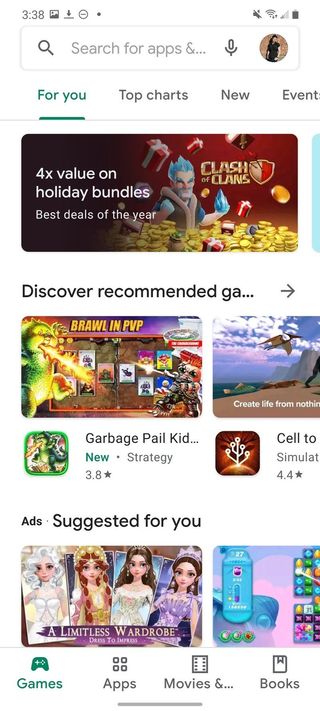This image is a tall, vertically-oriented rectangle, approximately twice as tall as it is wide, set against a white background with three distinct sections from top to bottom.

**Top Section:**
At the very top is a search bar. Directly below the search bar, there is a navigation menu with the following options: "For You" on the left, underlined in green, followed by "Top Charts," "New," and "Event" in gray text.

**Middle Section:**
Beneath the navigation menu, there is a prominent image. The background transitions from dark brown on the left to red on the right, featuring a light blue vertical bar to the right on the white background. The central focus of the image is a pile of gold coins stretching from the lower right to slightly past the middle. In the midst of the coins sits a cartoon figure with spiked blue hair, blue hands, blue eyebrows, and a vest with a tan collar. To the right of the character's head is the text "Clash of Clans." To the left of the figure, in white text, there are three lines: 
1. "4X value on,"
2. "Holiday Bundles,"
3. "Best Deals of the Year" (in slightly smaller text).

Below this prominent image, the white background contains text reading, "Discover Recommended GA..." with an arrow pointing to the right.

Further down, there are two side-by-side images; the first, larger image features a golden text reading "BRAWLNPVP" and depicts a green dragon with yellow chest and underside breathing fire. The background is a mix of various colors with indistinct square images. 

The second, smaller image has a purple sky with clouds, brown ground, green areas, gray mountains on the right, and a flying brown object. Underneath, in white letters on a brown background, it says "Create Life from Nothing."

Below this image is the text "Garbage Pail Kid..." Beneath this text, there's a green and yellow image on the left, an unrecognizable image in red and white to its right, followed by the text "CELL TO." Underneath, it says "new" in green, followed by a gray dot and "strategy" in gray text. Below "new" it indicates "3.8 star."

**Bottom Section:**
On a white background, below everything, black text reads "ads suggested for you." Under this, there is a cartoon image of four princesses, each in different attire:
1. On the left: a princess with white hair.
2. Next to her: a princess with long red hair.
3. Next to her: a princess with brown hair and a headdress.
4. On the right: a princess with brown hair wearing purple attire.

A purple banner across the bottom of the princesses reads "A Limitless Wardrobe" in white text. 

To the right is another image featuring a blue and pink background with various icons. 

At the very bottom, the section reads, from left to right, "games" with a game controller icon above it in green, "apps" with four squares above it, "movies and..." with a movie icon above it, and "books" with a book icon above it, all in gray text except "games."

The overall composition effectively segments different types of content, guiding the viewer through various features and offerings.